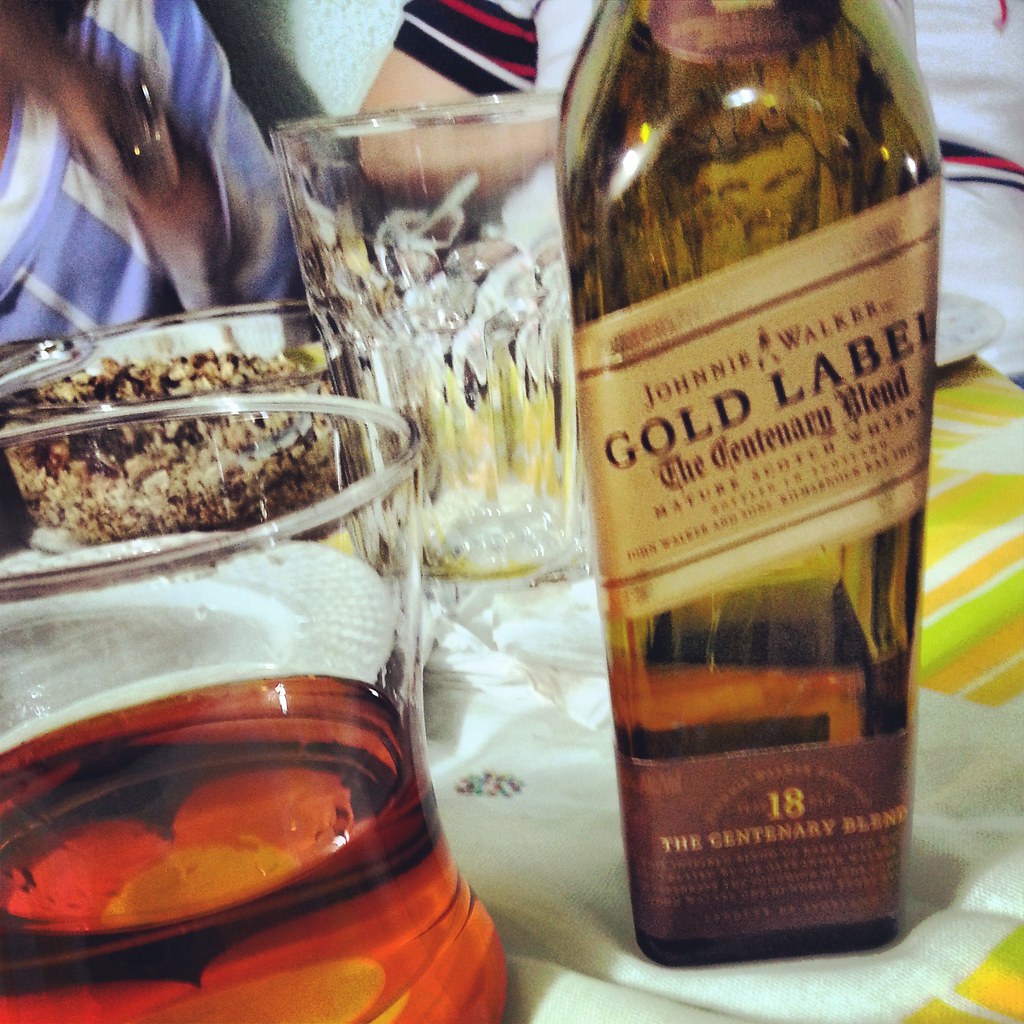This image is a close-up of a slightly blurry dinner table, likely taken in motion. The main focus is a distinctive gold square bottle of Johnny Walker Gold Label, The Centenary Blend, Mature Scotch Whiskey. The bottle's label, angled and golden with black text, prominently features the number "18" in white or gold on a brown section. To the left of this bottle, a squat glass filled about an inch with whiskey-brown liquid sits in extreme close-up. Behind the bottle, there's a taller water glass and a glass bowl containing brown, crumbly food, possibly grain. Additionally, a woman sits at the table, perhaps eating from the bowl, and silverware is faintly visible around the setting. The background suggests it's part of a larger dining scene, possibly on a tablecloth.